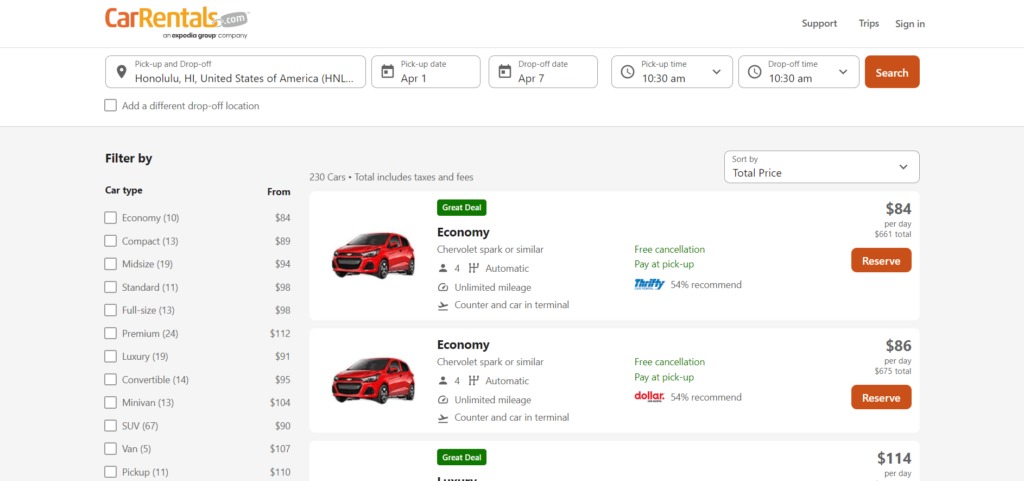The detailed screenshot features a large section of the Carrentals.com desktop webpage, offering a comprehensive view of their car rental search and filter interface. 

**Top Section:**
- **Logo and Navigation**: In the top left corner, the Carrentals.com logo is prominently displayed. On the far right, small grey letters read "Support," "Trips," and "Sign In."
- **Search Bar**: 
  - **Pick Up and Drop Off**: The left-most box, accompanied by a location icon, is set to "Honolulu, Hawaii, United States of America."
  - **Pick Up Date**: The adjacent smaller box displays "April 1st."
  - **Drop Off Date**: The next box to the right shows "April 7th."
  - **Pick Up Time**: The subsequent box indicates "10:30 a.m."
  - **Drop Off Time**: The following box is also set to "10:30 a.m."
  - **Search Button**: An orange "Search" button is positioned on the far right.

Below the pick-up and drop-off box on the far left, there is a checkbox, accompanied by small grey text that reads "Add a different drop-off location."

**Body Section:**
- **Filters**: On a grey background, the left side of the page is dedicated to filter options:
  - **Filter By**: Titled at the top.
  - **Car Type**: This section features clickable checkboxes for various car types, including "Economy," "Compact," "Midsize," "Standard," "Full Size," "Premium," "Luxury," "Convertible," "Minivan," "SUV," "Van," and "Pickup."
  - **From**: This section lists prices per day.

**Vehicle Listings**: 
- The main section on the right contains large white rectangular boxes, each featuring:
  - **Thumbnail Image**: On the left side of each box.
  - **Details**: Detailed descriptions to the right of the thumbnail.
  - **Pricing**: The far-right of each box displays the daily price at the top, with the total cost in smaller grey print below.
  - **Reserve Button**: An orange "Reserve" button is located at the far right of each listing.

Overall, this webpage layout efficiently displays essential search and filter features, along with detailed car rental options and pricing, all structured for user-friendly navigation and selection.